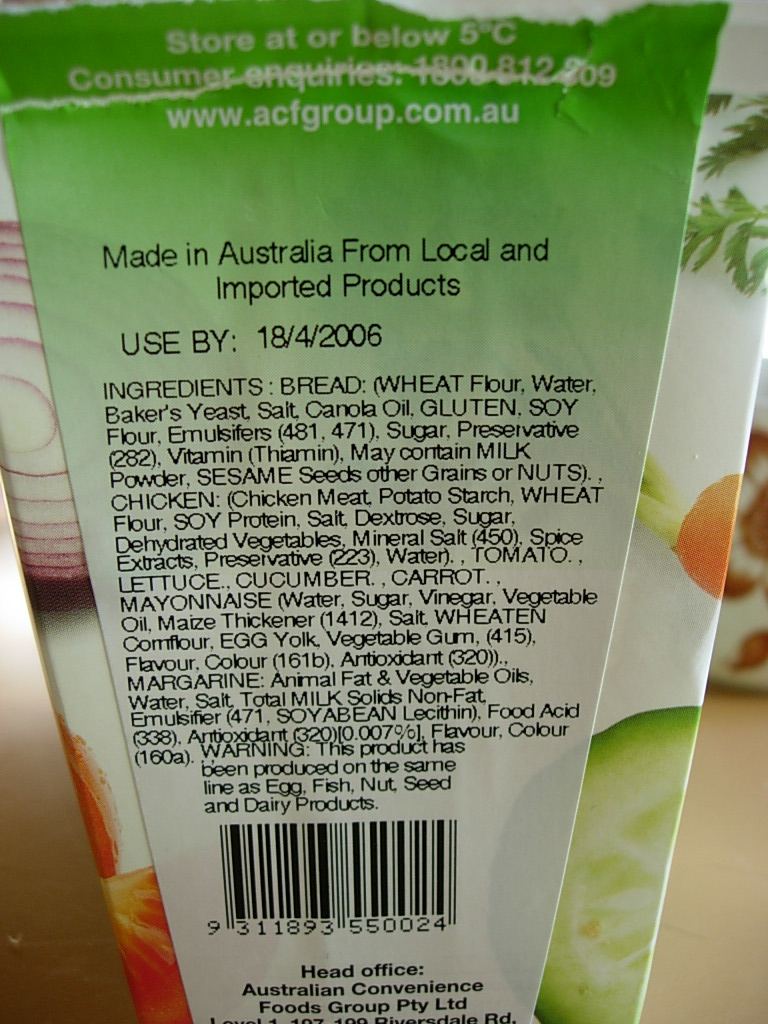This image shows a packaged food item from the Australian Convenience Foods Group. The label advises that the product should be stored at or below 5 degrees Celsius. The packaging contains bread, which is made from wheat and other ingredients, and includes chicken, though the exact nature of the product is unclear. The label is predominantly green, fading into white, with the text displayed on a white background. 

The label also includes a warning that the product has been produced in facilities that handle eggs, fish, nuts, seeds, and dairy products. There's a scannable barcode present as well. The background of the label features images of various vegetables, including onions, cucumbers, parsley, and red onions. The packaging is somewhat reminiscent of a milk container, though it obviously isn't that.

The entire setup appears to be placed on a counter.